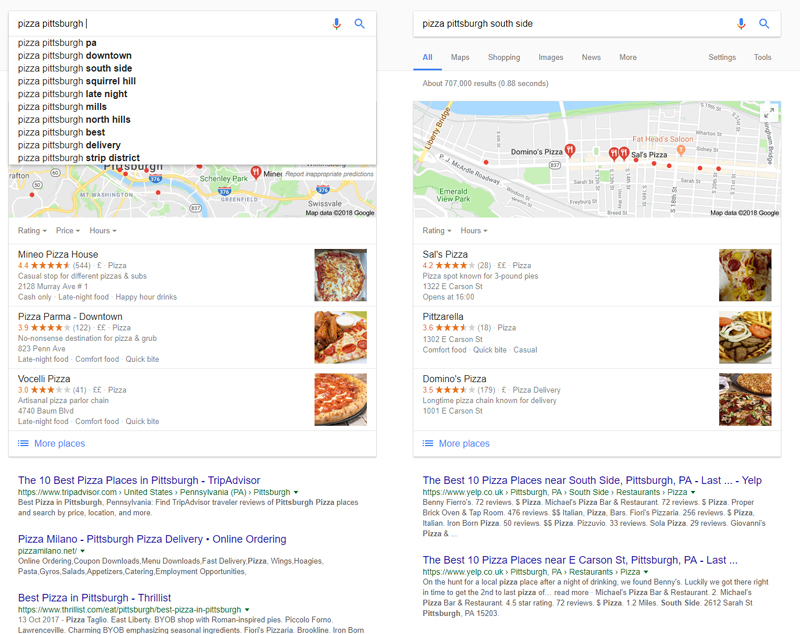This image shows a detailed search for pizza options in Pittsburgh's Southside. The scene captures someone typing "pizza Pittsburgh Southside" into a search bar. The search results feature a map prominently displaying various pins indicating pizza locations. The map includes interstates and side roads for easier navigation. Three highlighted pizza places are Mineo Pizza House, Pizza Parma, and Bocelli Pizza. 

On the right side, the search results provide actual photographs of the pizzas from these establishments, making the selection process more enticing. Additional information includes lists such as "The 10 Best Pizza Places in Pittsburgh" from TripAdvisor, "Pizza Milano Pittsburgh Pizza Delivery," "Online Ordering," and "Best Pizza in Pittsburgh" by The Thrillist. The search bar at the top clearly shows the query "pizza Pittsburgh Southside."

A more detailed section of the map is also visible, zooming in to show exactly where certain pizza places are located. Notable locations highlighted with red pins include Sal's Pizza, Pizzarella, and Domino's Pizza, all situated near a body of water. These locations also feature accompanying photographs showing their storefronts and interiors.

Beneath the map, there are related articles listing the "Best 10 Pizza Places Near Southside Pittsburgh" and "The Best 10 Pizza Places Near East Carson Street Pittsburgh," providing further recommendations for pizza enthusiasts in the area.